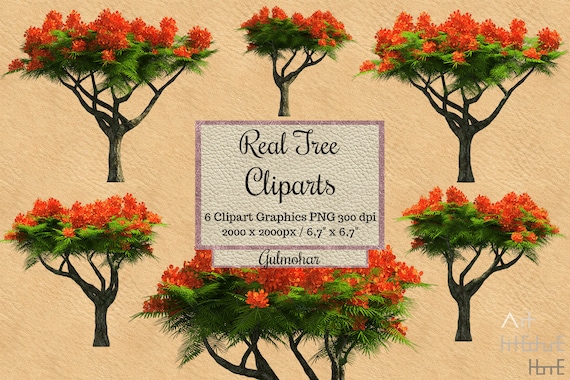The image is a detailed advertisement for RealTree Clipart. Set against a beige-pink background, the ad showcases six stylized tree graphics, each with brown trunks that branch outwards and upwards, displaying a verdant canopy of green leaves interspersed with red flowering buds at the very top. The trees' branches are bare below the canopy, focusing all foliage and blooms at the top. At the center of the layout is a prominent white box with a purple border containing text in black cursive font. This text provides details about the clipart package: "RealTree Cliparts. Six Clipart Graphics PNG 300 DPI 2000 x 2000 PX / 6.7 inches x 6.7 inches" and notes they are created by the author Golmahar. Additionally, there is a faint watermark in the bottom right corner featuring white and gray text, although it is not fully legible.